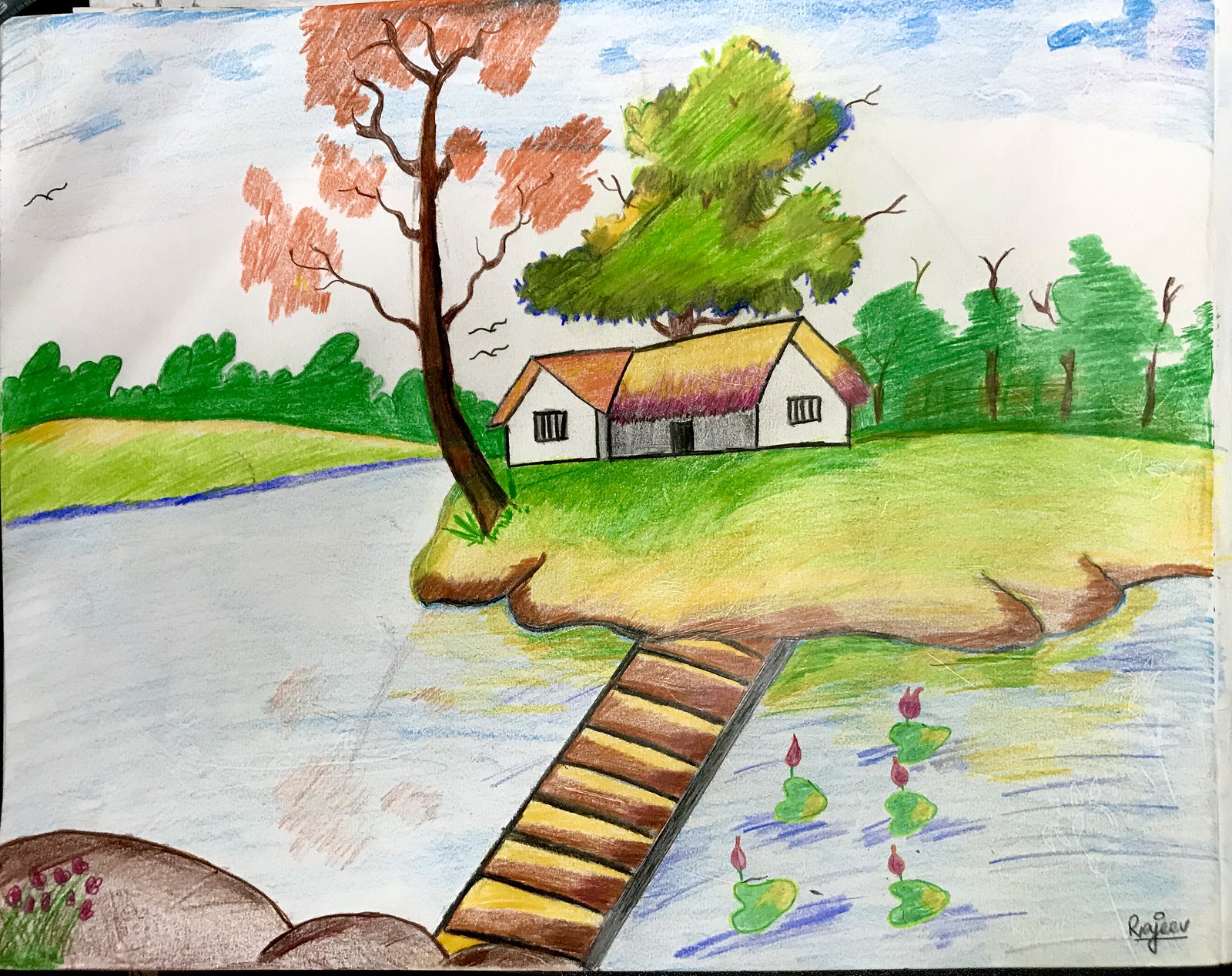In this colored pencil drawing, an enchanting scene unfolds featuring a quaint island nestled in a serene body of water. At the heart of the island stands a charming white house, crowned with a unique, two-tiered roof. The uppermost part of the roof appears to be crafted from hay, its yellow hue gradually transitioning to a purplish tint towards the edges, hinting at a change in light or material. Contrastingly, the left portion of the roof deviates from the hay-like design, adopting a more traditional V-shape with a flat, orange surface.

The house's structure includes a welcoming doorway and two windows, all set against its white façade. The house is situated on a lush green island, dotted with trees that boast vibrant foliage—some with striking pink leaves and others with the more traditional green.

In the background, a dense array of additional trees creates a rich tapestry of greenery. A wooden bridge, rendered in brown, connects the verdant island to an unseen shore, its planks leading the eye towards the serene oasis. Scattered in the surrounding water are five green lily pads, each adorned with delicate pink flowers, adding to the idyllic scene.

The bridge culminates in a small dark brown area on the island, peppered with charming pink flowers, rounding off this picturesque and tranquil depiction.